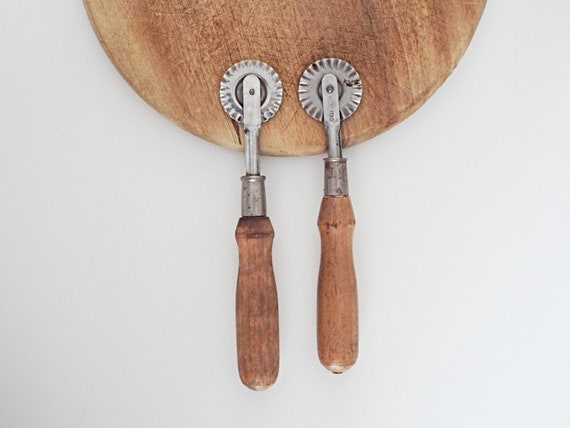In the simple, full-color photograph with a light gray off-white background, two pastry tools are prominently displayed. Each tool features a wooden handle of light brown hue, with the one on the left being slightly darker than the one on the right. The wooden part is attached to a metal segment that culminates in a textured rolling wheel used for making divots or decorative tracks on dough or pie crusts. These tools, which resemble dough cutters or crimpers, are positioned on a truncated circular wooden cutting board, which shares a similar color tone with the handles. The cutting board itself occupies the upper half of the image, with the pastry tools hanging off its bottom edge. The photograph appears to be carefully staged, possibly indoors, capturing the rustic aesthetic of the baking implements against the minimalist backdrop.